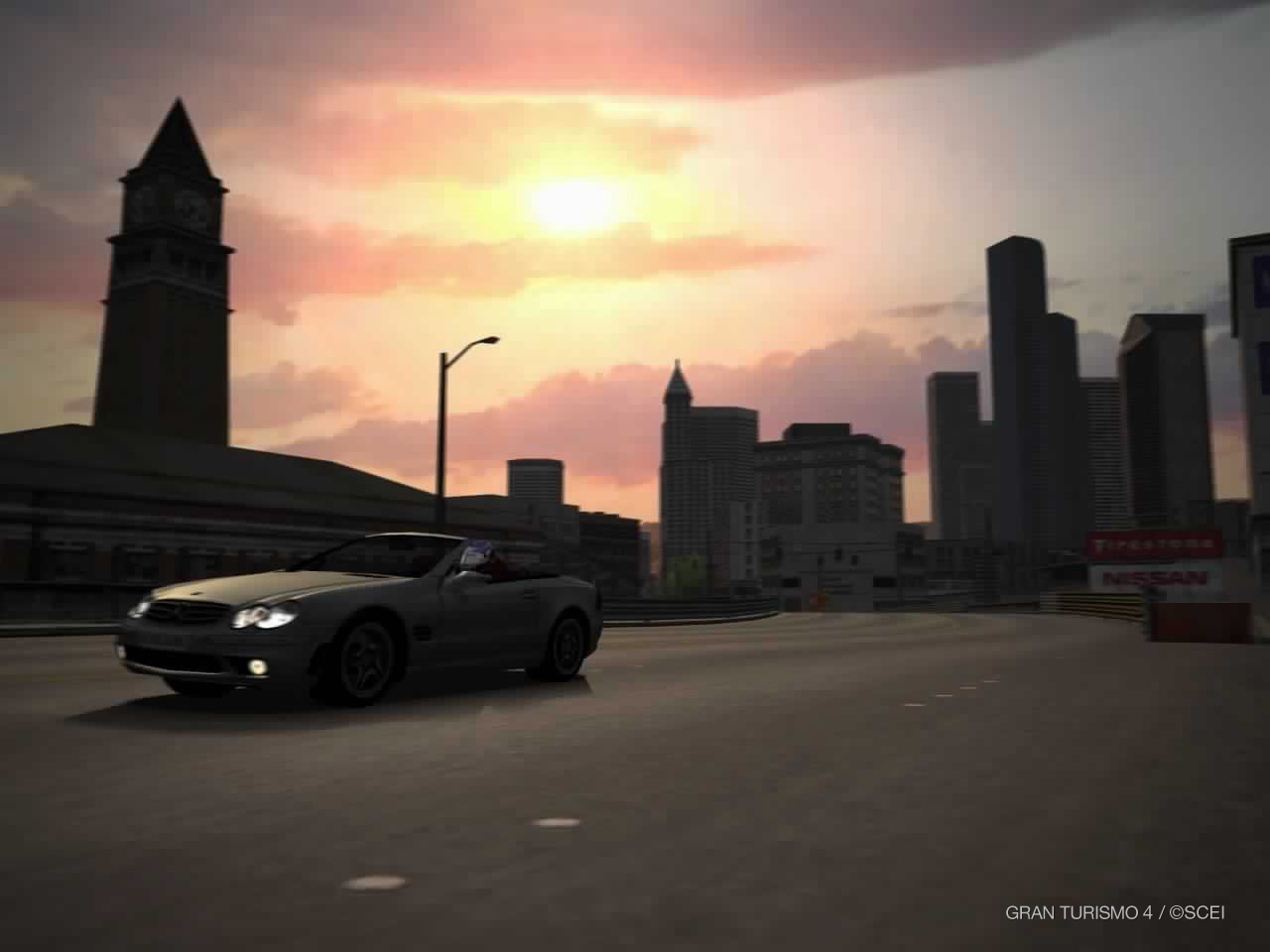A screenshot from the video game "Gran Turismo 4" captures a dynamic urban scene set under a grayish sky with patches of dense clouds. The sun, casting a faint yellow hue, peeks through the clouds, adding a subtle luminance to the scene. Dominating the left-hand side of the image is a towering building with a distinctive triangular top. On the opposite side, several large rectangular buildings contribute to the city's skyline. The foreground features a four-lane road, clearly demarcated with dotted lines indicating the lane divisions. In the upper left section of the road, a gray convertible with its headlights on is seen, suggesting a moment of active gameplay against the urban backdrop.